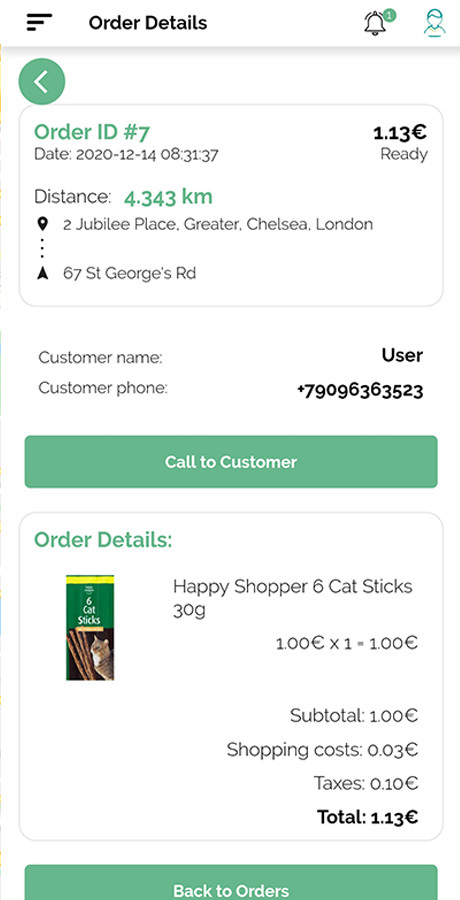In this image, a smartphone screen is displaying detailed order information within an e-commerce or delivery application. At the top of the screen, there is a notification bell icon with a red badge showing the number "1," indicating an unread notification. Next to it, there is an icon resembling a human silhouette, likely representing customer support or a live chat feature. Adjacent to these icons, horizontal bars suggest a menu option that, when clicked, provides additional navigational links to other sections of the app. A back arrow is also visible, allowing the user to return to the previous screen.

The main section of the screen provides comprehensive order details. The order is identified by ID number seven, with a timestamp of December 14, 2020, at 8:31:37. The total amount of £1.13 is specified, and the order status is marked as "ready." The delivery distance is noted as 4.343 kilometers to the destination at Jubilee Place, Greater Chelsea, London, specifically to the address 67 St. George's Road. The customer's name is listed as "user" along with a contact phone number: +7909-636-3523. A "call to customer" button is present for immediate contact with the customer.

In the detailed order summary, the item listed is "Happy Shopper Six Cat Sticks, 30 grams," priced at £1.00, with a quantity of one, leading to a subtotal of £1.00. Additional costs include a shopping fee of £0.03 and taxes of £0.10, bringing the total to £1.13. At the bottom of the screen, there is a "Back to Orders" button, allowing the user to navigate back to the main orders list.